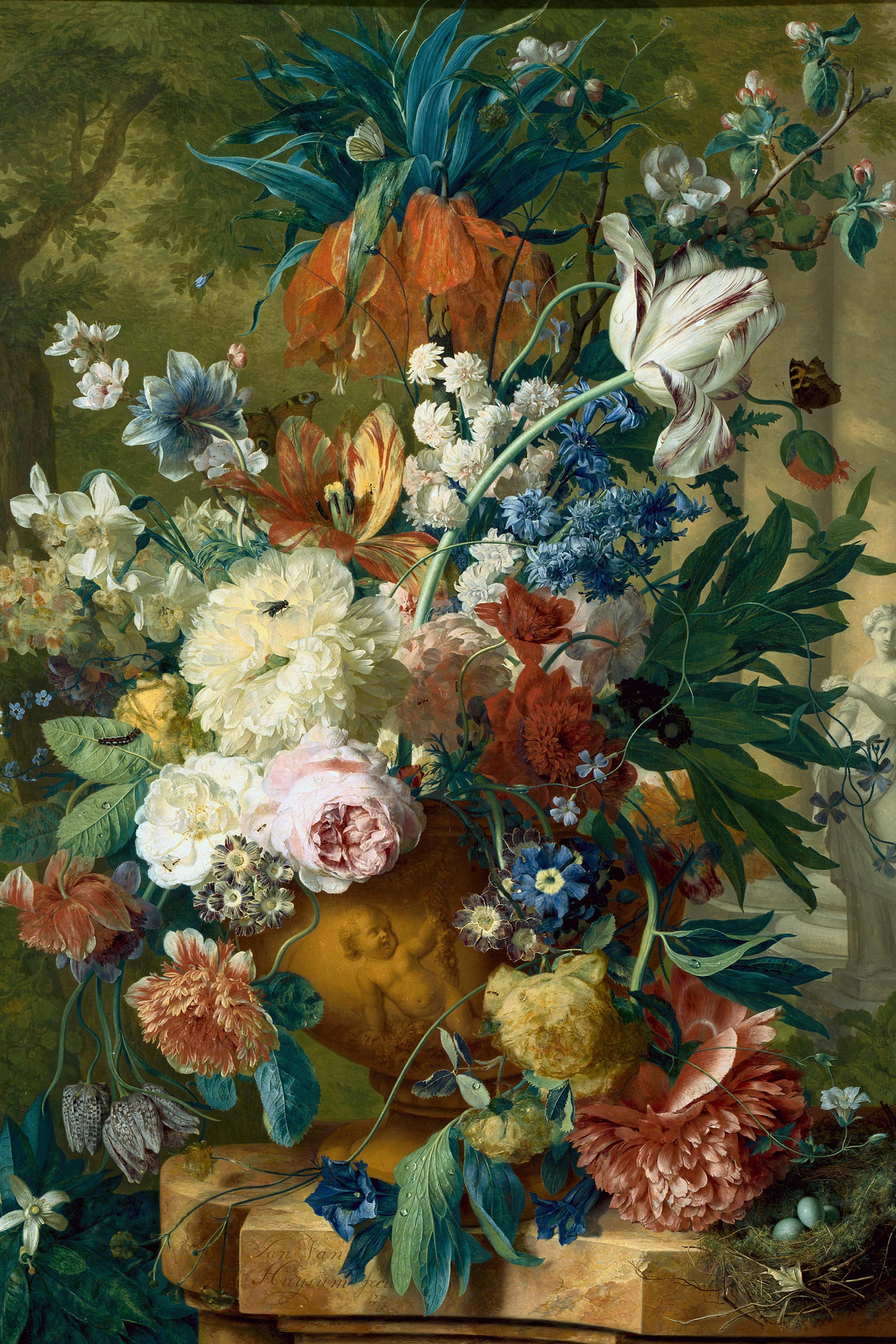This exquisite painting features a vibrant and colorful floral arrangement overflowing from an ornate, round, orange vase, adorned with a design of a child. The flowers, in a myriad of hues including pinks, oranges, whites, blues, lavenders, reds, and yellows, cascade in various directions, with some stretching upward and others bending forward. The vase is placed on a copper-colored pedestal and surrounded by lush green leaves. The backdrop presents a serene garden setting with a tree bearing green leaves on the left and a classical, white, Roman-style statue of a naked woman on the right. Notably, bird eggs nestled at the bottom right, along with an ornamental statue further enrich the background, adding depth and intrigue to the scene.